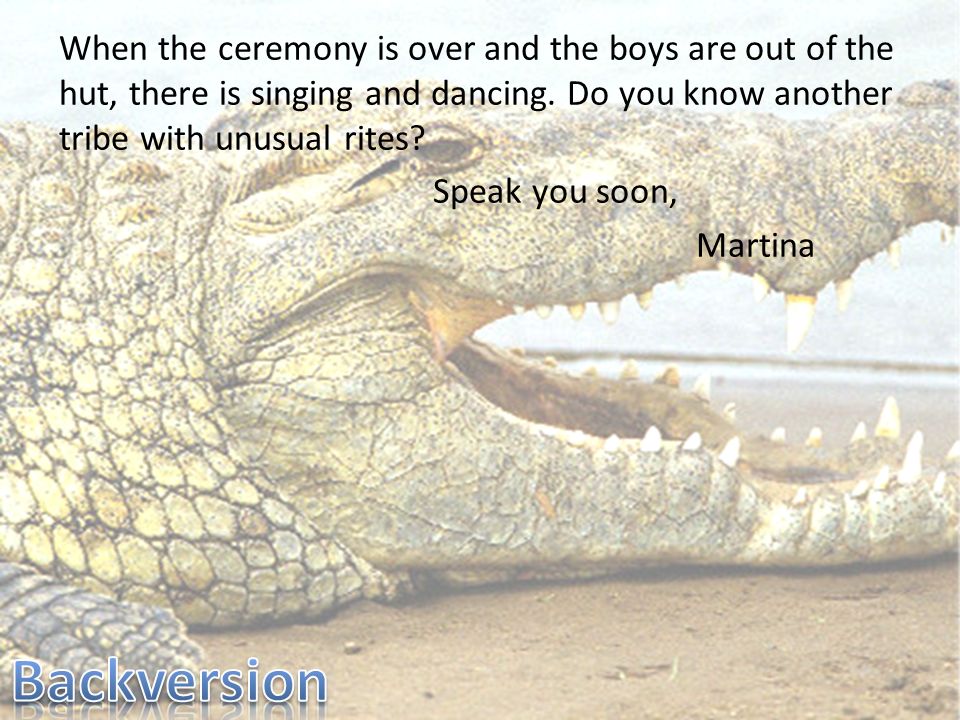The image depicts the head of a crocodile (or possibly an alligator) with its mouth open, facing to the right and revealing its sharp teeth. The animal is positioned on a shore, with brown dirt beneath it and the waterline behind its open mouth, giving the impression of a beach setting. The crocodile's head is slightly faded, with the background color of tan, brown, and gray hues contributing to the overall scene.

At the top of the image, in black writing, is the text: "When the ceremony is over and the boys are out of the hut, there is singing and dancing. Do you know another tribe with unusual rites?" This text extends over three lines. Further down in the middle of the image, it reads "speak to you soon," followed by the word "Martina" written slightly to the right, above one of the crocodile's prominent teeth and near its eye. In the bottom left-hand corner, the word "backversion" is displayed in blue lettering outlined in white. The photo appears to be taken outdoors during the daytime in a natural beach environment.